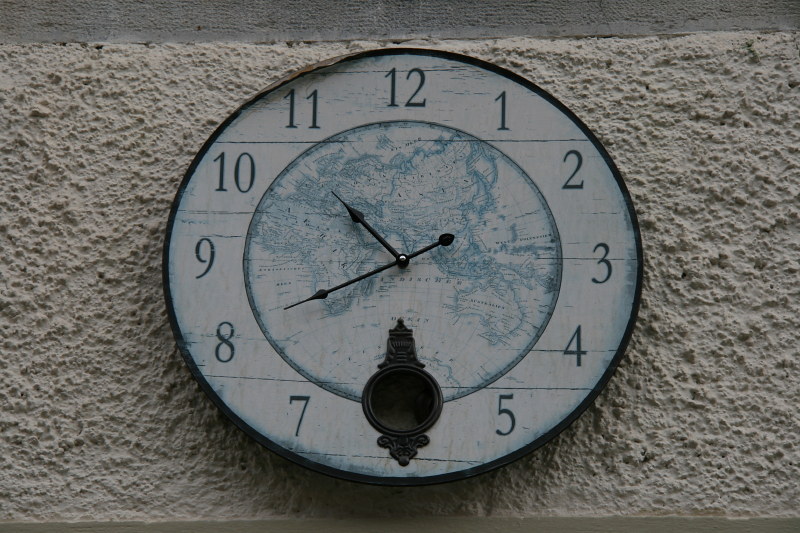An intricately designed clock with a unique face features a central circle that represents a map. The landmasses on the map are outlined in blue, while the areas signifying water are white, creating a stark contrast. This map is enclosed within its own circle. Surrounding this central map, another outer circle displays the clock numbers, which run clockwise starting from 12 and include 1, 2, 3, 4, 5, 7, 8, 9, 10, and 11, with the number 6 obscured. In place of the 6, there is an abstract element crafted from black pewter. The clock's two hands are also visible; the shorter hour hand is positioned between the 10 and 11, while the longer minute hand points to the 8.